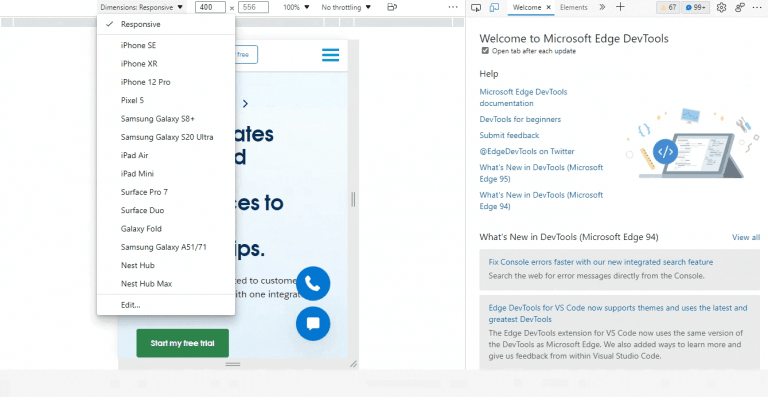The image features a dual-page screenshot showcasing a developmental tool interface on the left and a webpage on the right.

On the left side, the interface presents a page with a white background. At the top left corner is a drop-down menu with a dark gray header labeled "Dimensions: Responsive." The text is in dark gray. Beneath this header, the drop-down menu is light gray and lists multiple device emulation options, with "Responsive" checked and highlighted at the top. Following a thin gray separator line, the subsequent options from top to bottom are: iPhone SE, iPhone XR, iPhone 12 Pro, Pixel 5, Samsung Galaxy S8+, Samsung Galaxy S20 Ultra, iPad Air, iPad Mini, Surface Pro 7, Surface Duo, Galaxy Fold, Samsung Galaxy A51/71, Nest Hub, and Nest Hub Max. Another thin gray line separates these options from the "Edit..." option below.

Adjacent to the "Dimensions: Responsive" label, there are two input boxes for custom dimensions: the left box displays "400," followed by an "X," and the right box reads "556." To their right, it shows "100%" with a gray downward arrow, and "No Throttling" with another downward arrow beneath it. Below this setup, dark gray boxes obscure a light blue webpage with dark blue text, which is mostly hidden by the drop-down menu. Notably visible is a green button at the webpage's bottom left corner, featuring slightly rounded corners and white text reading "Start My Free Trial."

On the right side, the webpage has a white background with tabs at the top. One tab labeled "Welcome" is selected, appearing white with a blue underline and gray text, alongside a gray "X." The adjacent tab is labeled "Elements" and is in light gray, consistent with the rest of the header. The main content area below this header is titled "Welcome to Microsoft Edge DevTools."